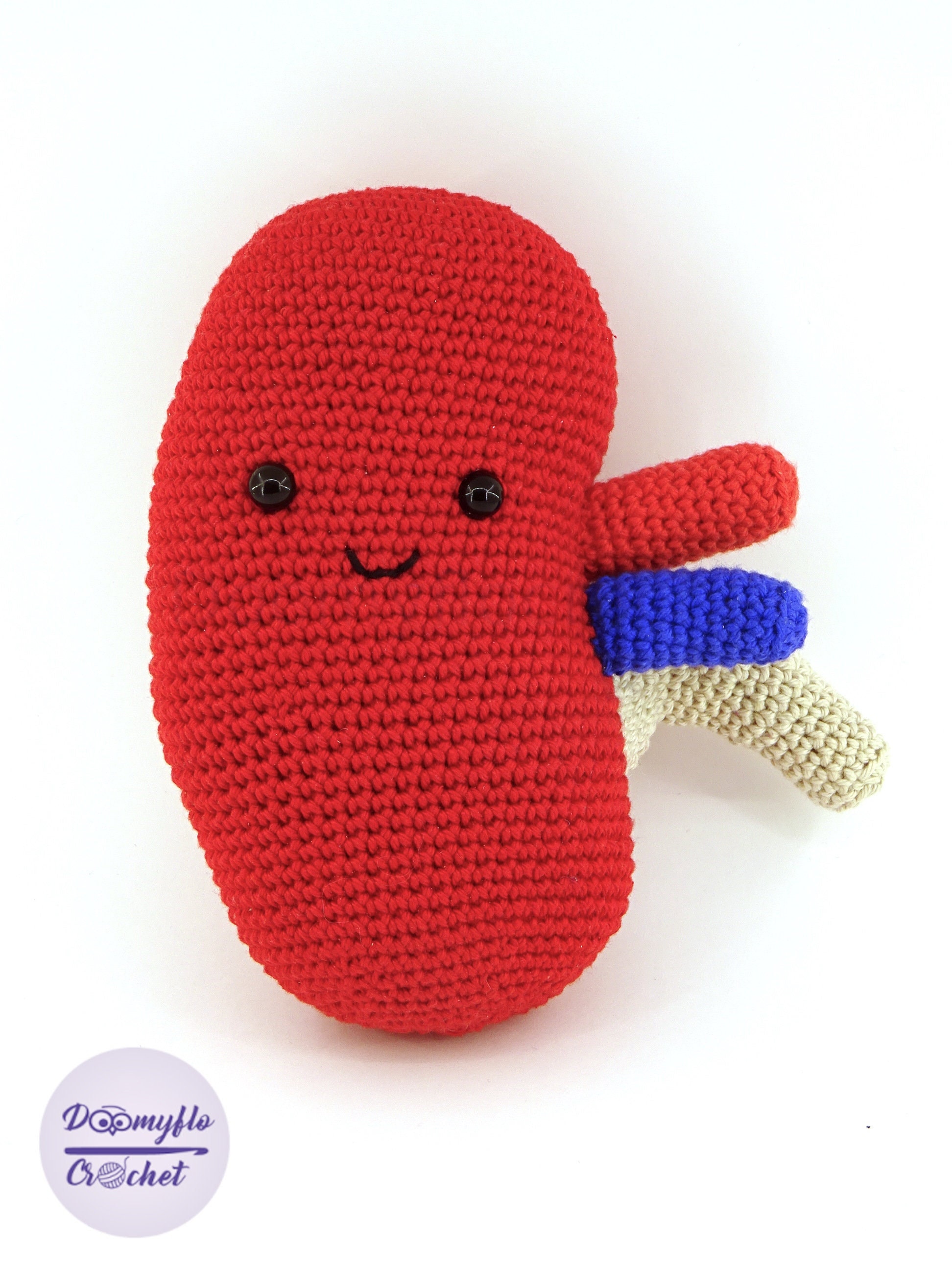The image is a photograph of a crocheted anatomical heart, designed with a playful, chibi style. The heart is primarily red and features three distinct extensions: a blue ventricle, a white ventricle, and another red ventricle. This whimsical heart has two small, black button eyes and a stitched, smiling mouth, giving it a charming and friendly appearance. The background is transparent white, suggesting the item is intended for sale or display. On the lower left-hand side of the image, there is a logo watermark that reads "DOO MYLLO Crochet," with the letters "O" replaced by eyes with beaks, adding a comedic touch. The crochet project appears to be small, roughly 7 to 8 inches tall.